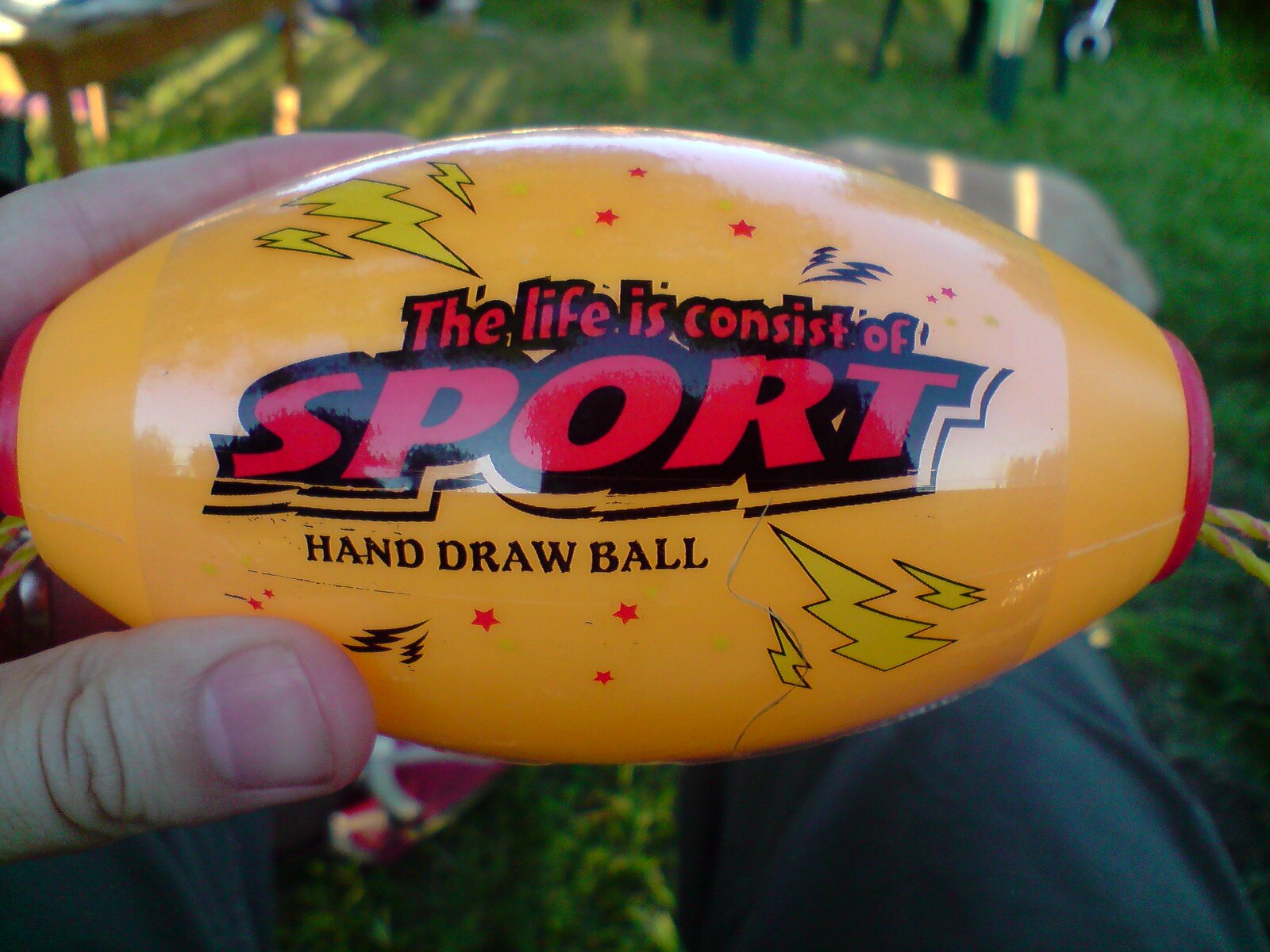This detailed close-up photograph features a Nerf-like football being held by a light-skinned person. The football stands out with its vibrant burnt orange body and striking red details. Across the football, in prominent red lowercase letters outlined in black, it reads "the life is consist of," followed by the word "SPORT" in large red capital letters, also outlined in black. Below this, there's a black outlined inscription in thin capital letters that states "hand-drawn ball." Complementing these inscriptions are several decorative elements: streaks of black lightning bolts, three prominent yellow lightning bolts, and multiple five-pointed red stars. 

The ball is held in the person's right hand, with their thumb and forefinger clearly visible, giving an idea of its size—approximately that of a hand, though perhaps slightly larger. In the background, the lush dark green grass contrasts with the person's green pants, adding depth to the scene. Also visible are shadows that suggest a relatively dim setting with some light filtering through. Partially glimpsed are other figures and a light brown table, though these elements are cut off and less defined.